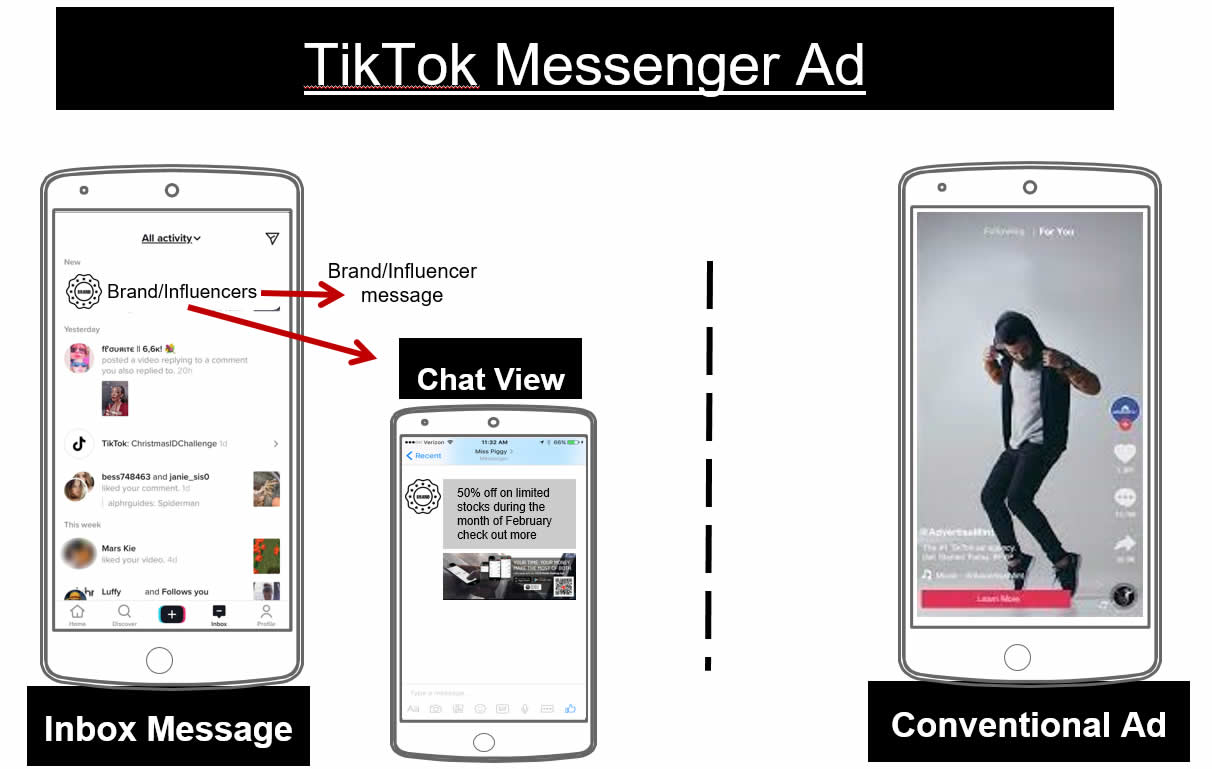The image features a promotional setup for Tick Tock Messenger, highlighted by distinct sections. At the top, a black bar with bold, underlined white text reads "Tick Tock Messenger Ad." Below it, a white bar separates the header from the main content. 

The main section presents three cell phones in a row. The center phone is noticeably smaller than the ones flanking it. The phone on the left is illustrated in black and white with text and symbols. It has "Brand Influencers" written on it, with red arrows pointing to labels that say "Brand Influencer Message" and "Chat View," the latter situated in a black box. This phone also features a "Chat View" duplicated on a smaller scale above it. At the bottom, another black box contains the text "Inbox Message."

A vertical dashed line demarcates the space between the left phone and the middle and right phones. The right phone mirrors the style of the left phone – black and white – but showcases a colored screen. On the screen, a lighter-skinned man with tattoos is depicted standing on his toes, knees bent, and hands tugging on his black hoodie. He wears a white t-shirt, black pants, and black shoes. Various Tick Tock icons adorn the screen. Below this image, "Conventional Ad" is written in white letters within a black box.

This detailed depiction contrasts the roles of brand influencers and conventional advertisements within the Tick Tock Messenger interface.